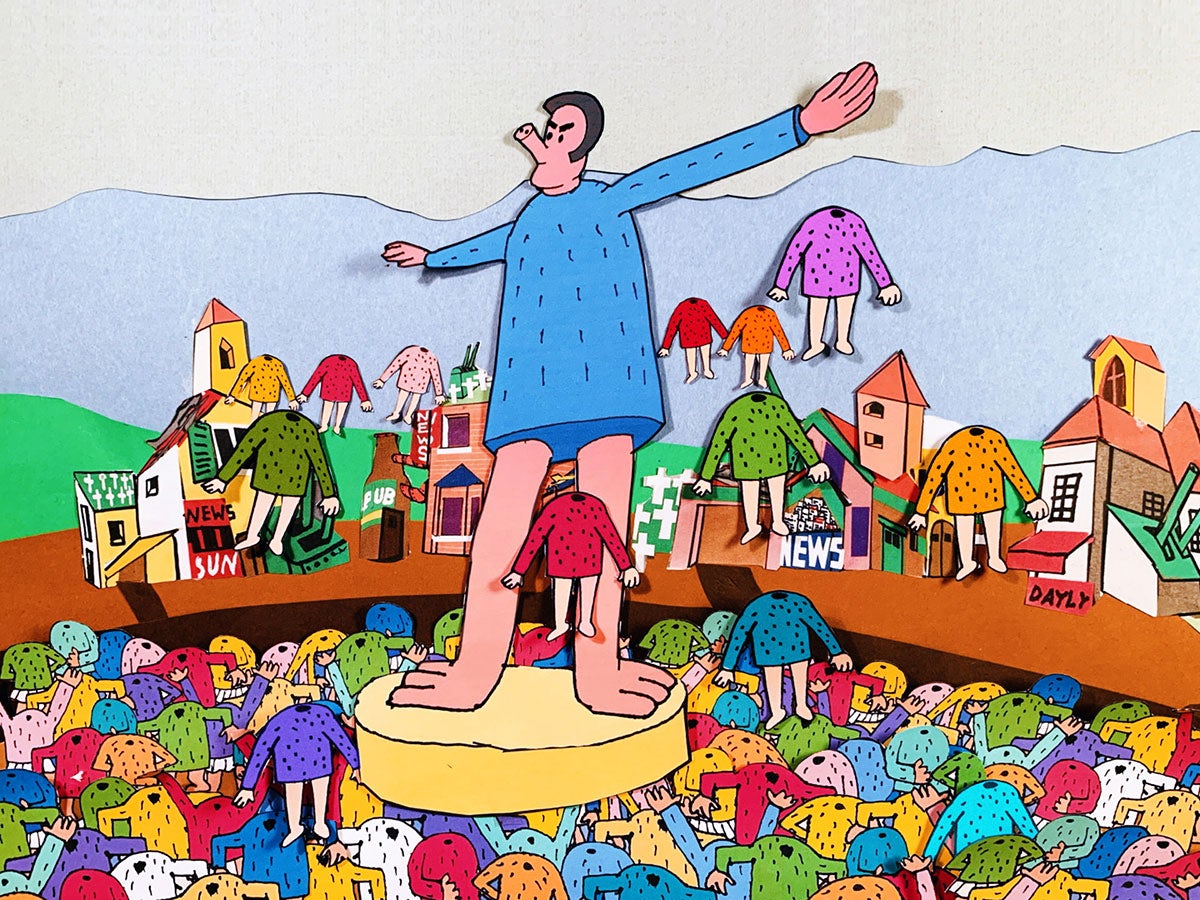The image is a detailed, cartoonish collage featuring a man with a pig snout. He has a human face with thick black eyebrows, two black dots for eyes, and reverse C-shaped black hair. The man is standing on a thick, yellow, coin-like circle, wearing a long-sleeved shirt adorned with little black lines. Below him, there is a pit filled with headless bodies dressed in colorful sweaters of various shades including purple, gray, yellow, white, and pink. The background showcases a small, curved city street lined with buildings labeled "Sun, news, and daily." Two pipes are emerging from a building on the right. The sky above is light blue with light gray cloud-like structures. Red and white crosses, suggesting a cemetery, are also visible in the distance. The scene is artistic and collage-like, with various cut-out elements and stickers adding to its surreal and vibrant composition.